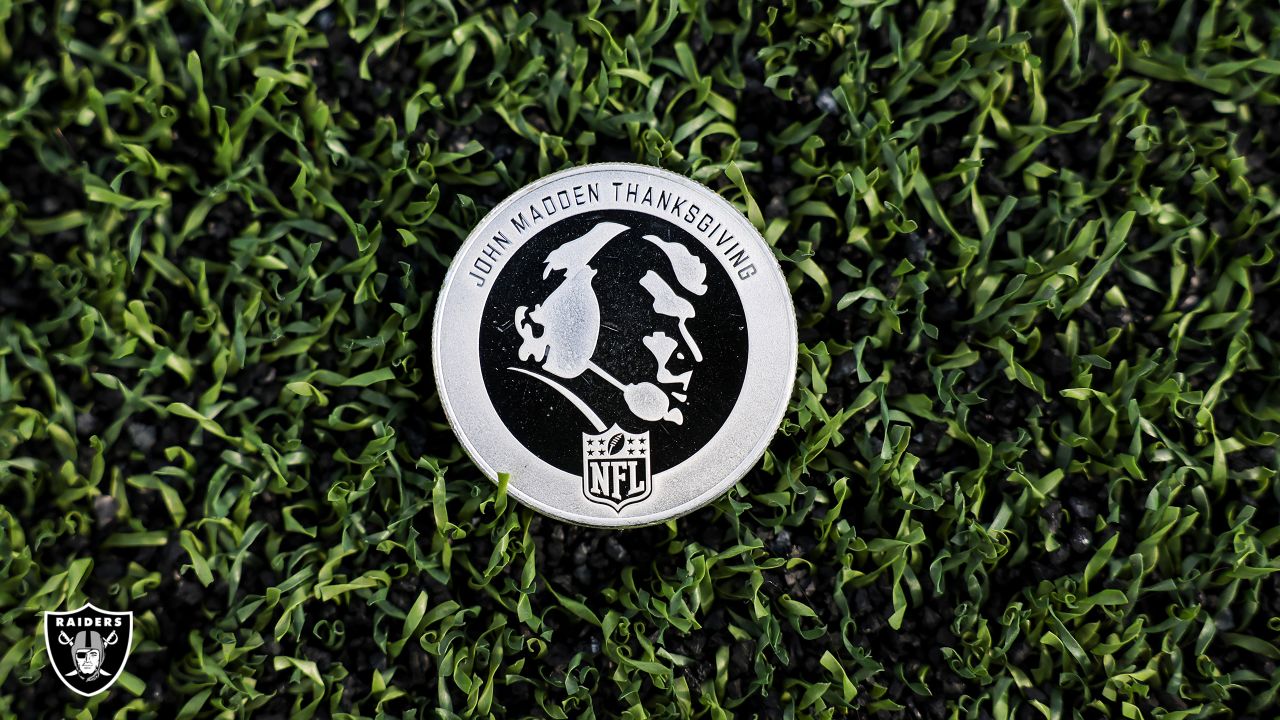The image displays a detailed silver coin prominently featuring a profile of John Madden, with the forward part of his face shaded in black and silver and traditional headphones with a microphone in silver. The inscription "John Madden Thanksgiving" is engraved above his image. The coin sits atop dark green AstroTurf, complete with black rubber pellets commonly found in NFL stadiums. In the lower left corner of the image is the Raiders' iconic black shield emblem, with a silver outline, showcasing a pirate head wearing an eyepatch with crossed swords behind it. Additionally, there is an NFL emblem with a football depicted at the bottom of the coin. The overall aesthetic of the image is dominated by the colors green, black, and silver, suggesting a promotional theme for the NFL or the Raiders.